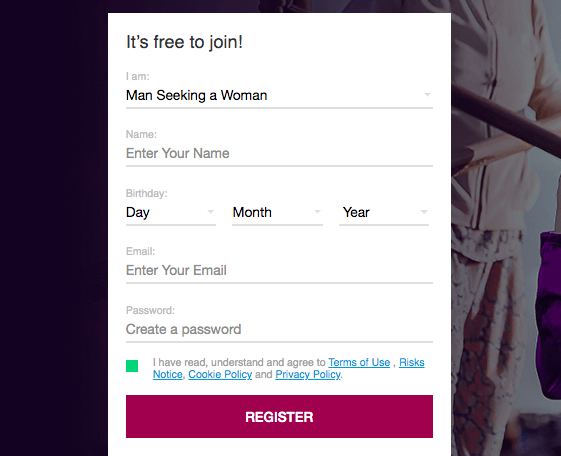A person stands against a dark background, dressed in a pink top and pink pants adorned with small gray designs. To the left of the individual is a rail, and a purple bag hangs from the edge of it. In the bottom right corner of the image, there is a small square. Dominating the center of the image is a large white box with text. The text reads, "It's free to join. I am a man seeking a woman." Below this, there is a line for entering details. A down arrow indicates fields for "Name" where users can enter their name, followed by a drop-down menu for "Birthday" comprising day, month, and year selections. Further down are fields for "Email," where users can enter their email, and "Password," where users can create a password. Towards the bottom, there is a green checkbox next to the text stating, "I have read, understand, and agree to the Terms of Use, Risk Notice, Cookie Policy, and Privacy Policy," with clickable, underlined blue links for each policy. Finally, a purple box marked "Register" signifies the registration button.